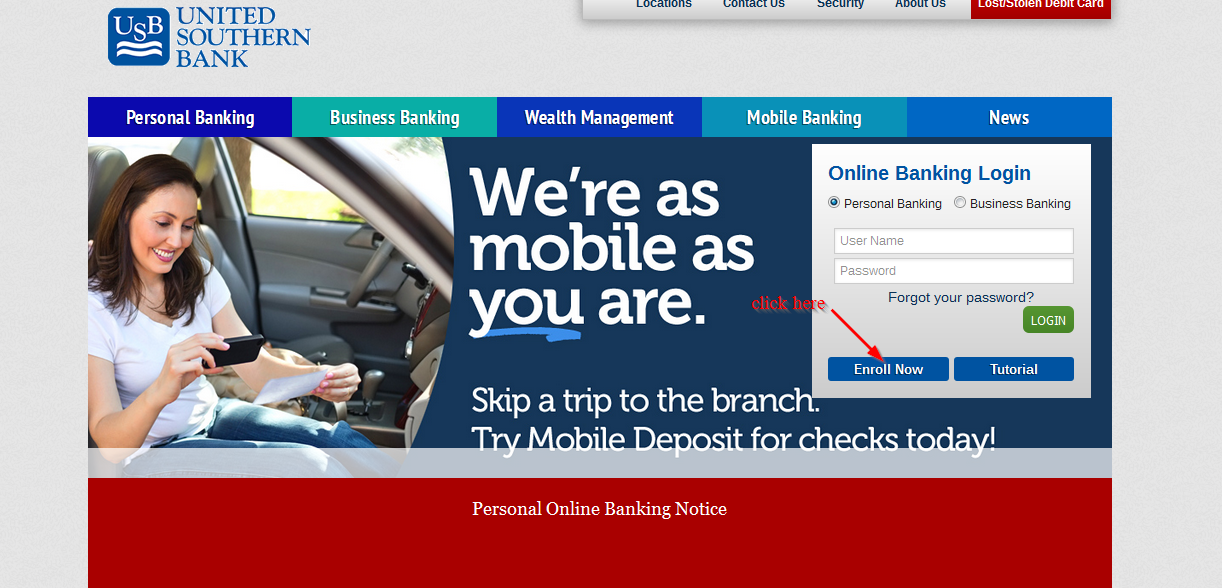Description: This is a detailed screenshot of the United Southern Bank's (USB) opening web page, showcasing its various components and features targeting its users.

In the upper left-hand corner, the blue square logo with white text "USB" features two white wavy lines beneath it, symbolizing United Southern Bank. Directly to the right, in stacked blue text, reads "United Southern Bank".

In the upper right portion of the screen, there is a comprehensive menu bar including options for "Locations," "Contact Us," "Security," "About Us," and a prominently displayed red button labeled "Lost/Stolen Debit Card."

Moving down the page, a large rectangular section is adorned with a red, white, and blue theme. Across the top of this section are clickable tabs for different services: "Personal Banking," "Business Banking," "Wealth Management," "Mobile Banking," and "News," all designed in shades of blue and teal.

Centrally, a visually engaging advertisement and login section span the width of the page. An image features a woman with long brown hair, wearing a white t-shirt and blue jeans, sitting in a sedan. She is smiling while holding a check and taking a photo of it, suggestive of mobile deposit functionality. Accompanying this image is the slogan in white text: "We're as mobile as you are," followed by, "Skip a trip to the branch, try mobile deposit for checks today."

Adjacent to this visual, on the right, is the "Online Banking Login" box, composed of a white square with options to select either "Personal Banking" or "Business Banking". It includes fields for a username, password, a "Forgot Your Password" link, and a green "Login" button. Additional links for "Enroll Now" and a tutorial are also present, with a red "Click Here" arrow pointing towards the "Enroll Now" button, indicating a step-by-step instruction page.

Finally, at the bottom quarter of the screen, a large red rectangular section presents an important notice in white text: "Personal Online Banking Notice."